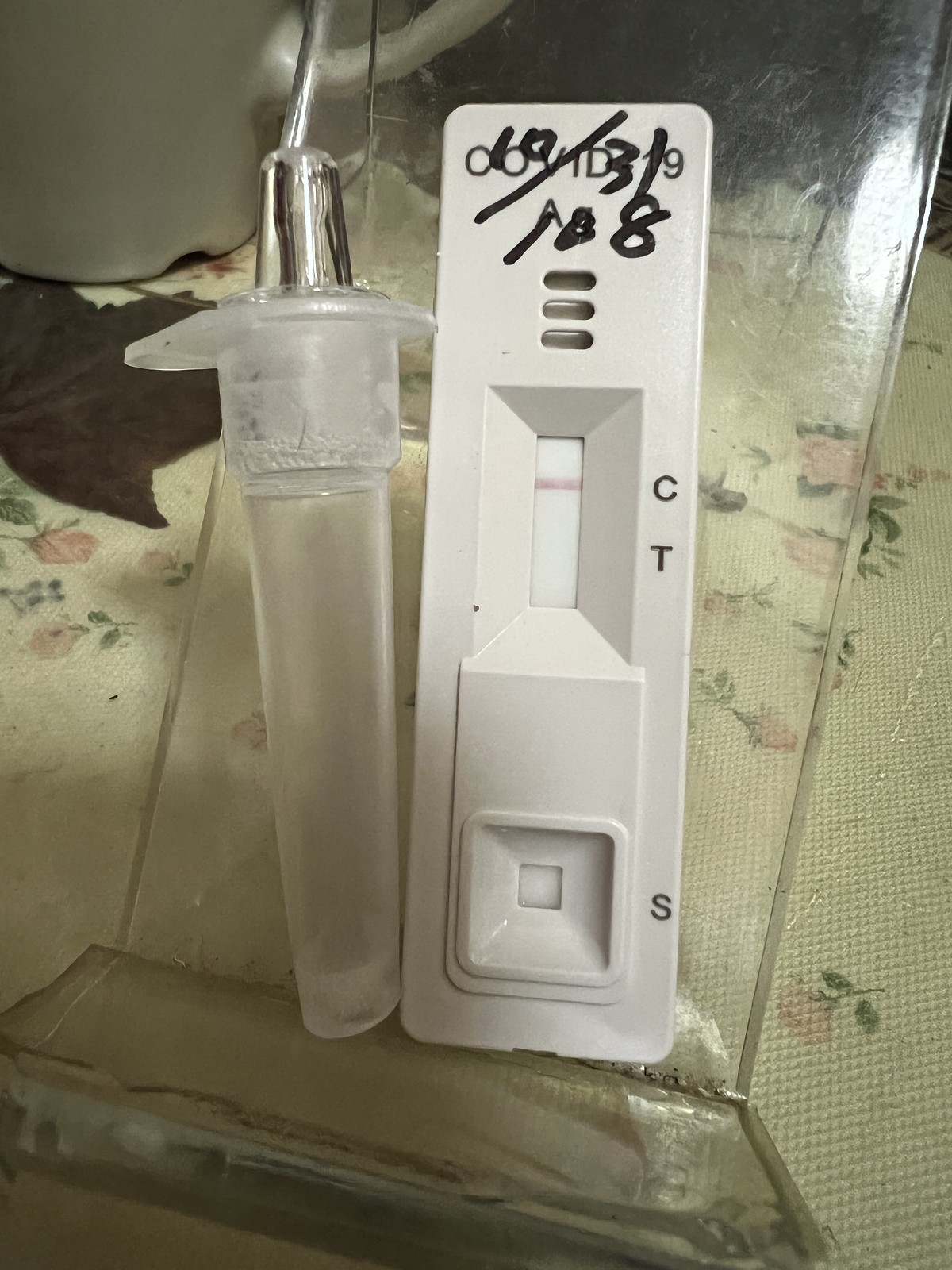The photograph showcases a negative COVID-19 test placed on a clear acrylic stand, reminiscent of a cookbook stand. It is positioned on a tablecloth adorned with delicate rose patterns. The white plastic test, approximately a few inches long, displays a pink control line indicating a negative result. At the top, "COVID-19" is printed, and the date "10/31" along with the number "108" are handwritten in bold, black Sharpie. Accompanying the test is a tube, likely used for the nasal swab, capped with a dropper lid. In the background, a white ceramic mug with a handle is visible, along with a dark olive-green leaf, possibly a grape leaf, lying beneath its edge.